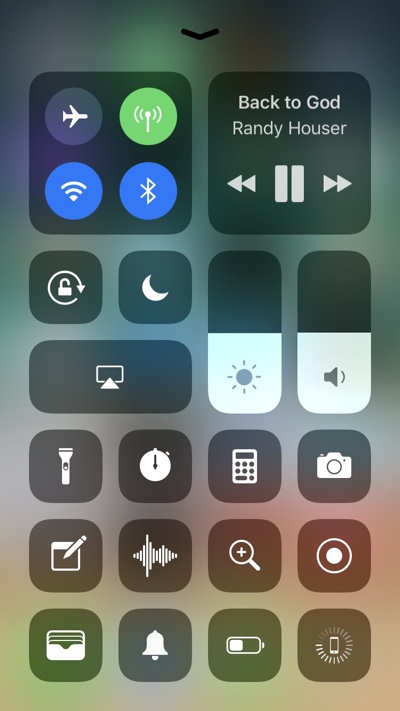This image is a detailed screenshot of a smartphone's home screen, capturing various control icons and music information. 

At the top left, there are icons for essential settings like Airplane Mode, Wi-Fi, and Bluetooth. The right side prominently displays the text "Back to God, Randy Houser," indicating the user is currently listening to this song. 

Beneath these settings, there are additional icons for various tools: flashlight, volume control, calculator, camera, notes, and an alarm clock icon, suggesting options for alarms or timers. The battery life indicator is also visible, along with an icon for adjusting the screen backlighting. 

The overall background of the screenshot is a grayish color, with all the icons neatly positioned inside dark gray boxes and rendered in white for clear visibility.